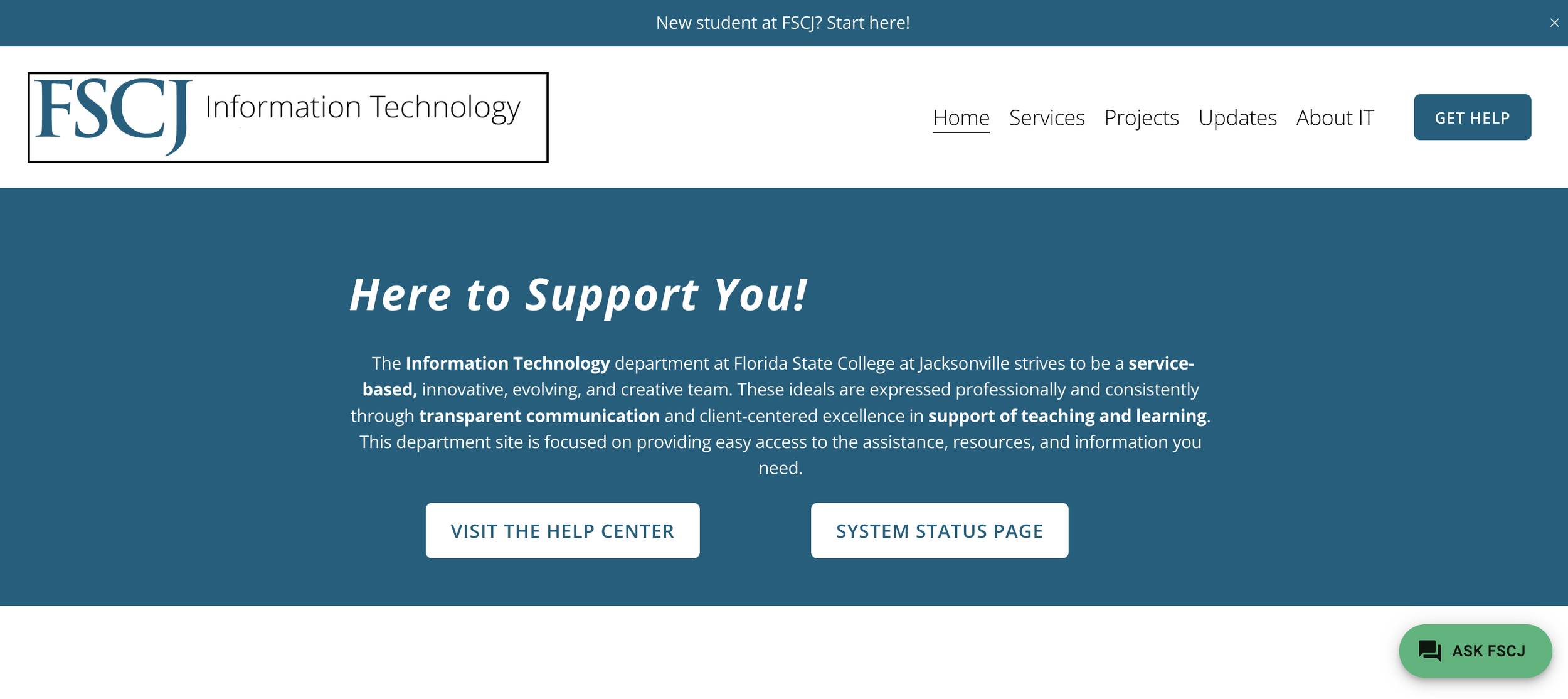The web page features a dark blue header and bezel, creating a unified color theme at the top of the page. Centrally positioned in the header is white text that reads, "New Student at FSCJ? Start Here!" with a white 'X' located on the far right. Below the header is a large off-white rectangle with grey undertones, which contains another bordered rectangle aligning with its left edge. This inner rectangle has a black border and matches the dark blue background color.

Within this bordered section, the text "This is FSCJ" is displayed prominently in bold blue letters, followed by "Information Technology" in black text. To the right, various navigational tabs are listed in black text: "Home," "Services," "Projects," "Updates," and "About," with "Home" being selected and underlined in black.

Towards the bottom, there is a clickable rectangular button with a dark blue background and white text that says "Get Help." Underneath that, in a dark blue section, the page states in bold white text, "Here to Support You!" Beneath this proclamation, additional white text reads, "The Information Technology Department of Florida State College at Jacksonville strives to be a service-based, innovative, evolving, and creative team. These ideals are expressed professionally and consistently through transparent communication and client-centered excellence in supportive teaching and learning."

The webpage aims to provide easy access to needed assistance, resources, and information. It includes two white background buttons with dark blue text at the bottom: "Visit the Help Center" on the left and "System Status Page" on the right. Lastly, in the lower right corner is a dark green oval icon with black chat boxes and the text "Ask FSCJ" beside it.